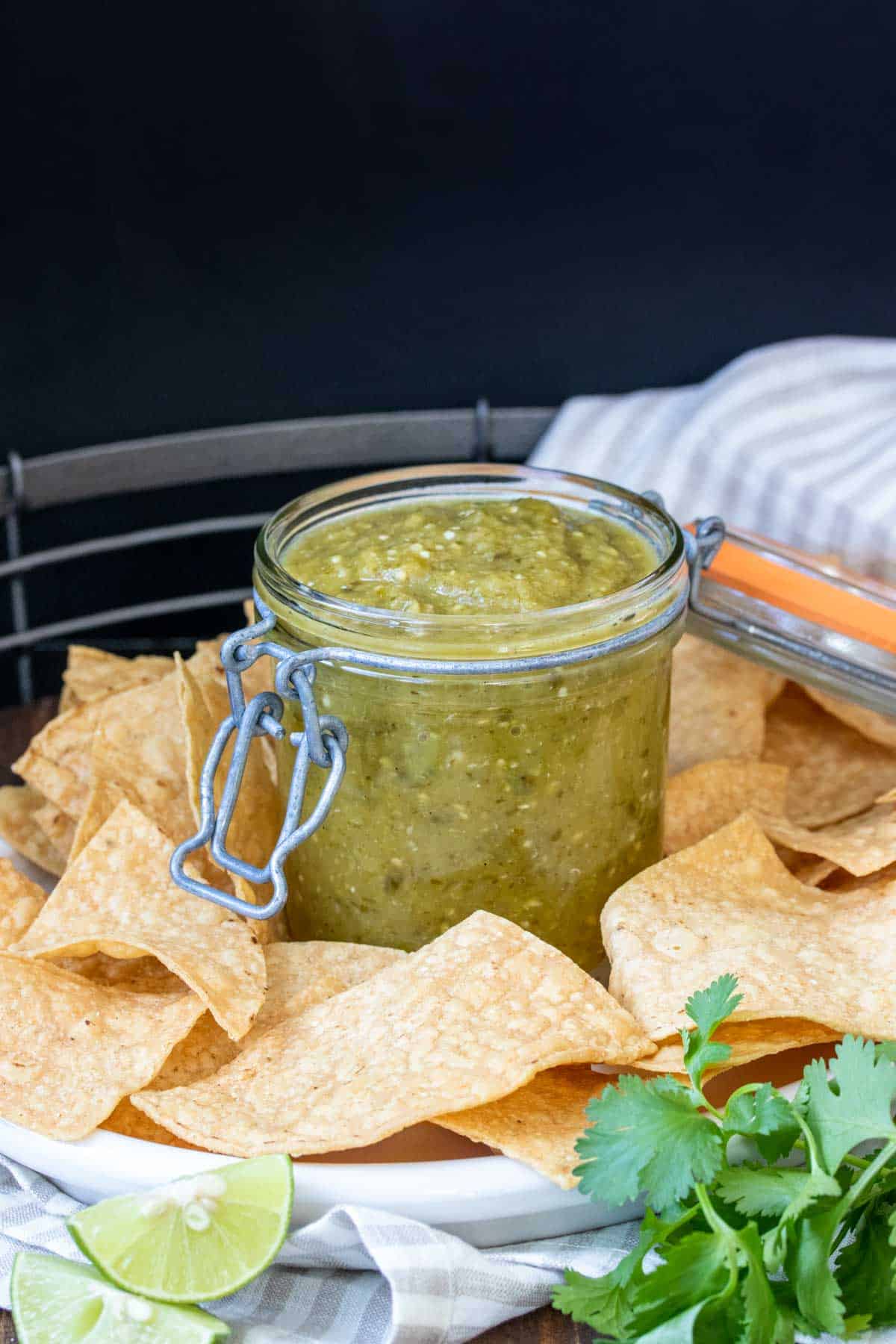In the foreground of the photograph, a pristine white plate hosts an inviting arrangement of golden-brown tortilla chips, each crisply textured and replete with rustic ridges. Central to this appetizing tableau is a small, glass mason jar, carefully propped open, and generously filled with chunky green guacamole, its surface flecked with various seasonings. Surrounding this jar, the tortilla chips beckon with their crunchy allure.

Complementing this visual feast, the lower left corner of the plate features two bright, light green lime slices, seeds visible at their center, ready to add a zesty twist. To the lower right rests a delicate bunch of thin, fresh cilantro, its vibrant green leaves adding a touch of herbal freshness.

The setup is presented against a navy blue backdrop, possibly a wall, which subtly contrasts with the white and gray striped fabric lying below the ensemble, creating a harmonious color balance. This detailed depiction captures the essence of a well-prepared appetizer tray, inviting and rich in visual texture.